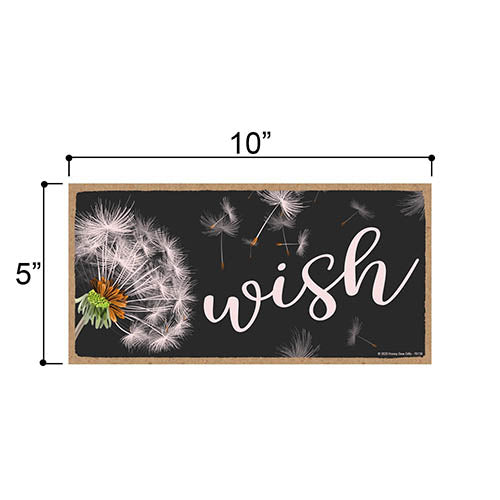An image depicts a 10-inch by 5-inch decorative chalkboard with a rustic, unfinished wood border set against a white background. The blackboard features the word "wish" written in whimsical, white cursive script. Adjacent to the word on the left side, a detailed, zoomed-in dandelion is illustrated, with its seeds elegantly drifting away across the board. The dandelion displays varying colors, including green at the base and subtle brown tones where the seeds disperse. A small copyright symbol is visible in the bottom right corner, accentuating the board's artistic authenticity.